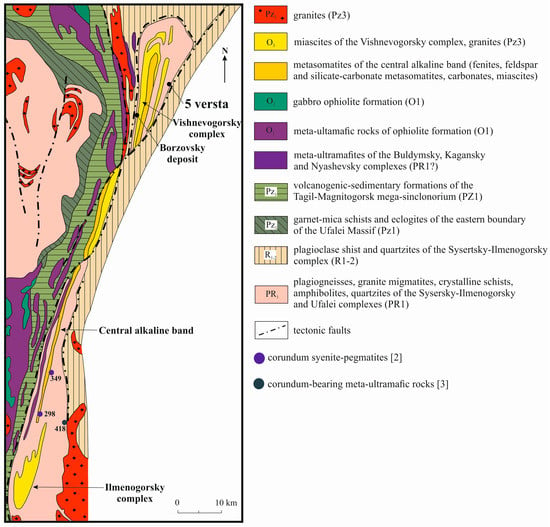The image is a detailed vertical diagram, likely a geological map, featuring a spectrum of colors including tan, pink, yellow, red, green, and purple, all meticulously labeled. The top of the diagram has an arrow pointing up, marked with an "N" for north, indicating orientation. Each color and shape on the map corresponds to different geological formations and structures, with a comprehensive legend to the right explaining the symbols. For instance, red areas denote granites, while yellow areas indicate miascites. Various shades of purple correspond to meta-ultramafic rocks of ophiolite formation, and white sections represent tectonic faults. The map also includes names of geological complexes and deposits like "Vishniv Gorski complex Borzovski deposit" and "Ilmeno Gorski complex." Additional symbols such as a purple dot and a dark green dot are also explained in the legend, which aids in understanding the precise geological makeup depicted in the map.